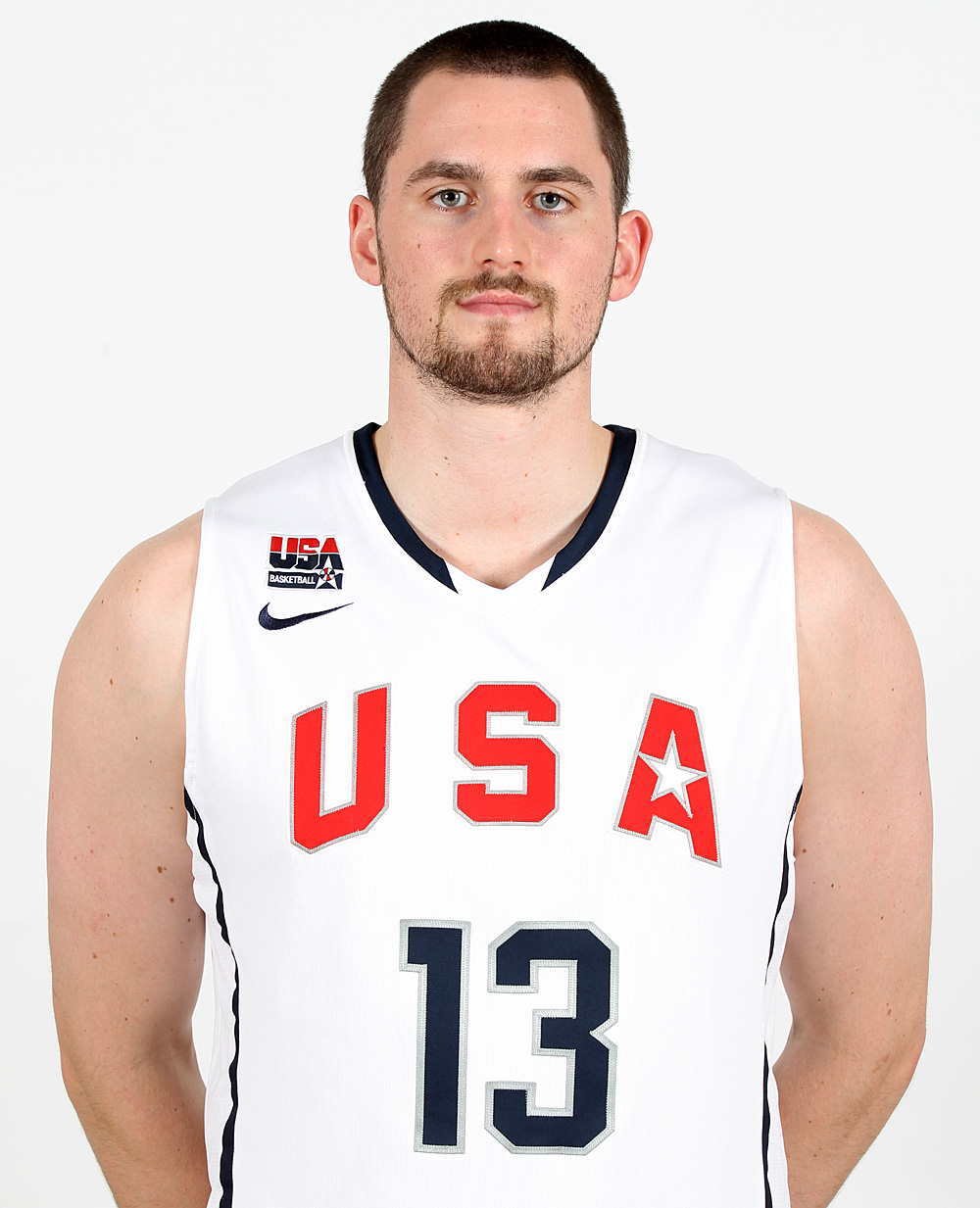This image features a Caucasian athlete standing in front of a blank white background in a promotional photo. He has a buzz cut with brown hair and his facial hair consists of a goatee that connects slightly to the sides of his face. His eyes have a greenish-blue hue, and he is staring directly at the camera with a serious expression. The athlete is wearing a white sleeveless jersey with blue collar trim and blue stripes on the sides. The jersey prominently displays "USA" in red lettering with a star in the center of the letter “A,” and the number “13” in blue underneath, both outlined in silver. On his right shoulder, there is a logo that reads "USA Baseball" with a star at the end, split into red and blue halves, and a small Nike logo beneath it. He stands with his hands behind his back, emphasizing his focused and composed demeanor.